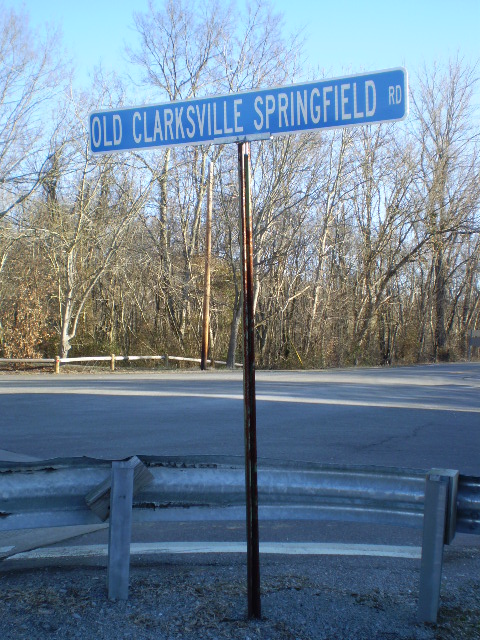In the photograph taken during a bright and sunny day, we see an intersection featuring a street sign that reads "Old Clarksville Springfield Road." The sign is attached to a blue and white pole positioned at a street corner. The corner itself is graveled and encircled by a curved metal barrier. Across the intersection, the scene is dominated by a dense array of bare trees, casting shadows across the road. The streets, marked with white lines, appear deserted, with no vehicles in sight. Additional details include yellow poles visible across the street and the overall ambiance accentuated by a clear blue sky.